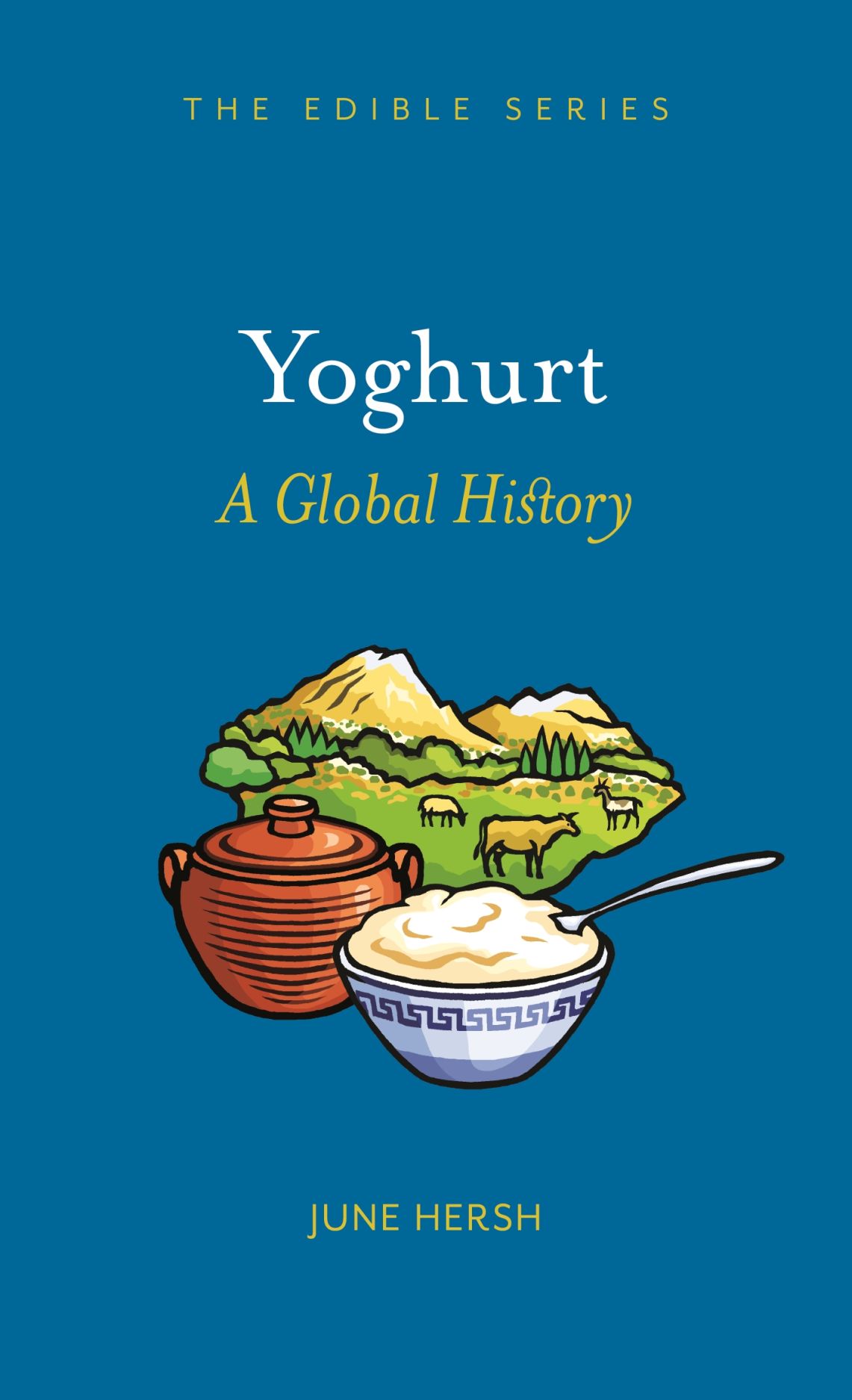This is a cover image of a book titled "Yogurt: A Global History," part of The Edible Series. The background of the cover is a solid blue. At the top, golden text reads "The Edible Series" in an all-capitals, sans-serif font. Below that, "Yogurt" is prominently displayed in white, serif font, followed by "A Global History" in italicized gold, serif font. 

The central illustration depicts a farm scene with lush green fields, grazing cattle and horses, and a backdrop of mountains. Additionally, there are green trees scattered throughout the landscape. Featured prominently in the foreground are two bowls: one filled with yogurt and decorated with a white and purple pattern, and the other, a reddish-brown closed pot. At the bottom middle of the cover, the author's name, June Hirsch, is written in gold, sans-serif font. The overall design is simplistic yet detailed, effectively capturing the essence of the book's subject matter.